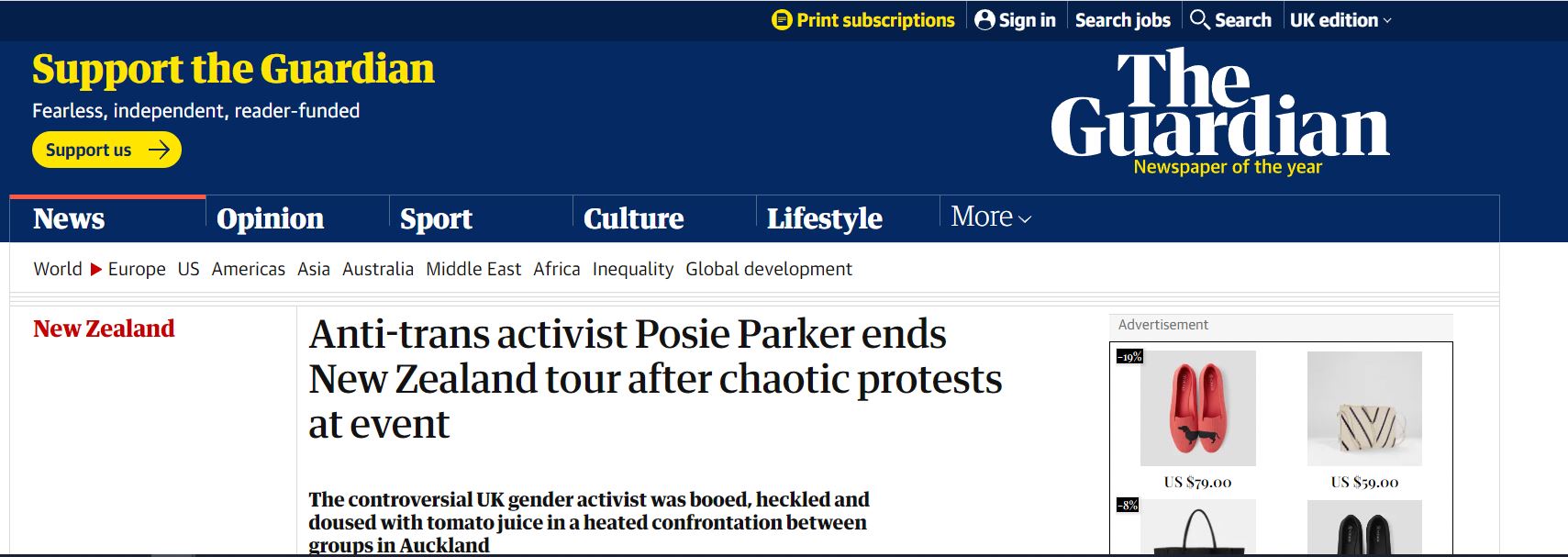This image is a screenshot of a news article from The Guardian's website. The interface presents a plethora of elements designed for navigation and user engagement. 

At the top-right corner, options such as "Print subscription," "Sign in," "Search jobs," and the "UK edition" are available for readers. Adjacent on the right side, the webpage prominently displays "The Guardian" in white typography, accompanied by a yellow banner declaring it "Newspaper of the Year."

On the left-hand side of the page, a yellow call to action urges readers to "Support The Guardian," emphasizing its ethos of being "Fearless, independent, reader funded."

Below the header, the main navigation menu spans from left to right, including categories like "News," "Opinion," "Sport," "Culture," "Lifestyle," and a dropdown for more options. In red text, the word "New Zealand" is visible on the left sidebar, indicating the article's regional focus.

The main focus of the page is the headline of a news story: "Anti-trans activist Posey Parker ends New Zealand tour after chaotic protests at event." This headline is prominently displayed in large black letters at the central bottom of the image. Accompanying the headline, a subheading elaborates that "The controversial UK gender activist was booed, heckled, and doused with tomato juice in a heated confrontation between groups in Auckland."

On the right side of the image, there is an advertisement displaying various pieces of clothing, including red shoes, a purse, another purse, and another pair of shoes.

The overall composition combines essential content with navigational tools and promotional elements, all within The Guardian's recognizable design framework.